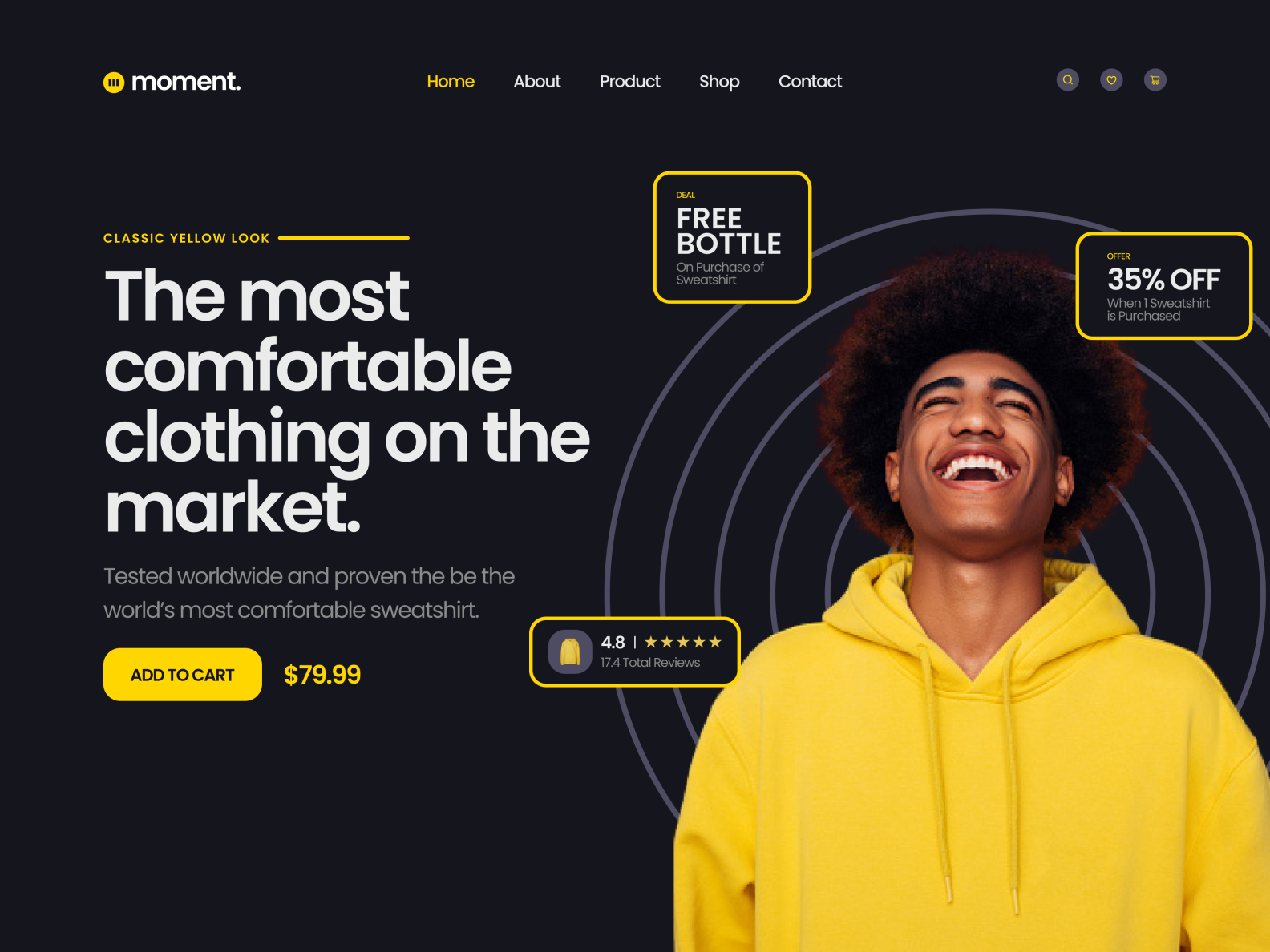This screenshot from the Moment website showcases a vibrant yellow hoodie priced at $79.99. Despite the relatively high price, the product boasts an impressive 4.8-star rating from 17.4 total reviews and is currently available with a 35% discount. In the bottom right corner of the screen, a digital image features a person modeling the brightly-colored sweatshirt, highlighting its eye-catching hue and stylish design. An enticing offer for a free bottle is also prominently advertised on the site. The overall webpage design utilizes a sleek black background with contrasting yellow and white font for enhanced readability and visual appeal.